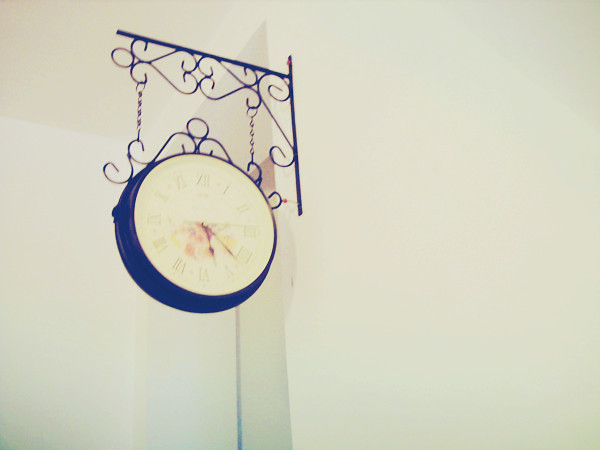This photograph captures a striking wall clock prominently mounted on a plain white wall. The image is characterized by high brightness, illuminating the intricate details of the clock. The clock is affixed high up on the wall, supported by an ornate black iron frame that projects outward before curving gently downward. The clock is suspended from this frame by two sturdy, black chain links, enhancing its elegant presentation.

Adorning the clock itself is a black border featuring an intricate swirly pattern, adding to its decorative appeal. The clock face is a crisp white, embellished with delicate red and yellow floral motifs that bring a touch of color to the monochromatic scheme. The time is marked by Roman numerals, which stand out clearly against the elaborate backdrop, making the clock not only a functional timepiece but also a decorative statement.